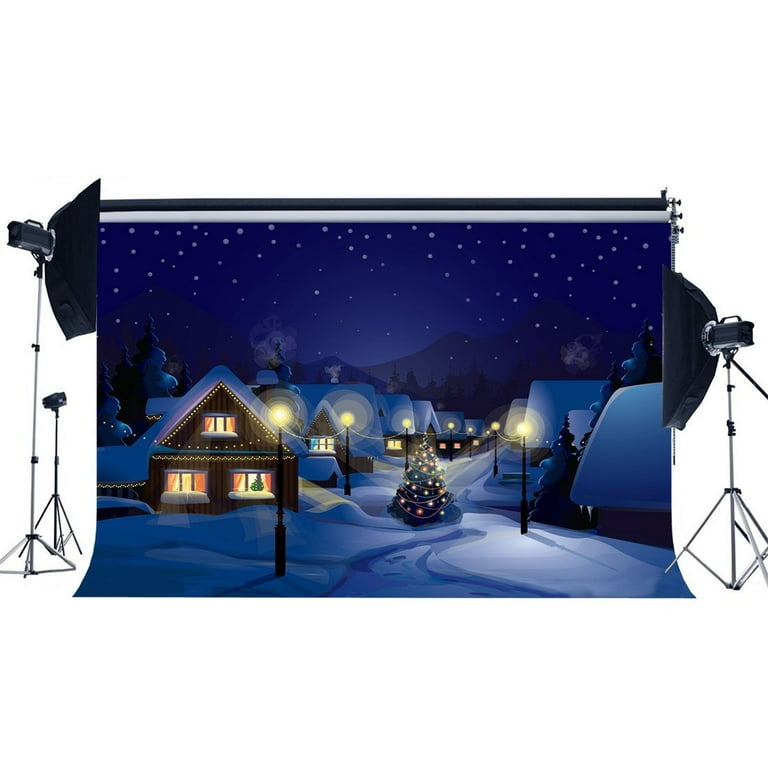This AI-generated photograph features a horizontal rectangle composition showcasing a detailed, festive Christmas scene. The main focus is two large screens on stands at the center, displaying an AI-generated snow-covered village scene. Flanking the screens are two studio lights on stands, with an additional smaller tripod or easel positioned behind them. The scene on the screens appears to be a backdrop, suitable for holiday-themed photo shoots, depicting a quaint winter village at night.

In the foreground of the scene, small brown wooden chalets are adorned with Christmas lights, particularly one A-frame cottage with a steep roof, single lit window on the roofline, and two lower windows. The village street beneath is blanketed in snow, complete with grooves indicating foot or vehicle traffic. A single, decorated Christmas tree stands proudly in the center, while globe-shaped street lamps, draped with twinkling Christmas lights, line the street. The atmosphere is set against a blue-toned, starry night sky with falling snowflakes and silhouettes of mountains in the backdrop. The overall effect evokes a charming, wintry Christmas village, ideal for capturing nostalgic holiday photographs.